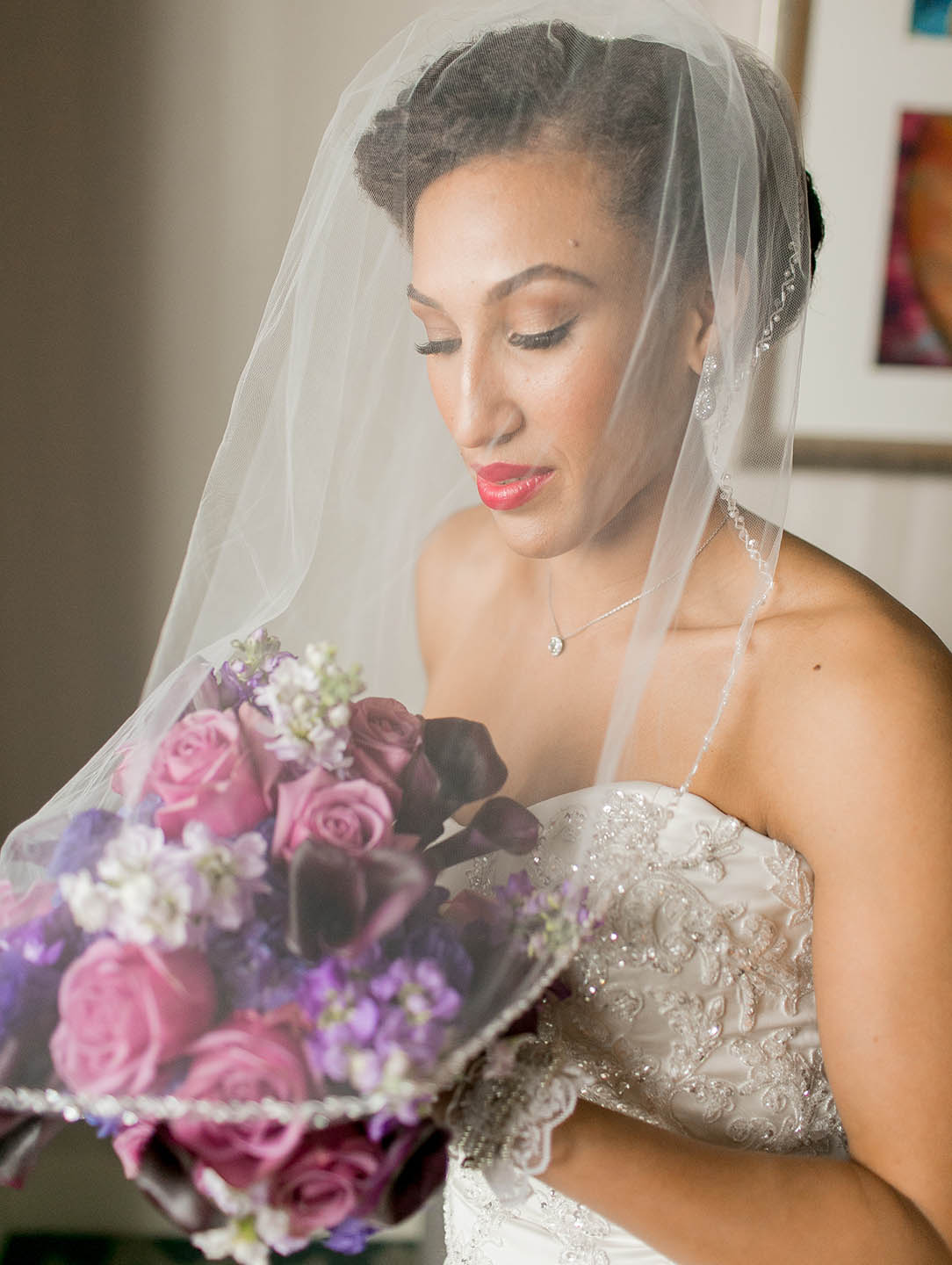In the photograph, a light-skinned Black woman, who appears to be a bride, is captured moments before her wedding. She has her eyes gently closed or potentially looking downward, exuding a serene and contemplative expression. Adorned in a strapless wedding gown with intricate lace appliqué and a beaded bodice featuring a sweetheart neckline, she epitomizes bridal elegance. Covering part of her face is a sheer veil, adding a layer of mystery and tradition. Her hair is styled in an elaborate updo, possibly braided or twisted, complementing her sophisticated look.

She wears a thin, delicate silver necklace with a clear gemstone, drawing subtle attention to her neckline. Her makeup includes striking red lipstick, and her long lashes accentuate her closed or downward-cast eyes. The bride's hands are elegantly holding a bouquet of mixed flowers, including pink and dark purple roses, lavender flowers, and hints of white florals, adding a burst of color to her ensemble.

The background behind her is beige, with a visible framed photograph featuring a white mat and sections of red, blue, and orange, enclosed in a wooden or gold frame, contributing an artistic touch to the scene. Her overall appearance, combined with the intricate details of her dress and bouquet, encapsulates a moment of poised anticipation before her nuptials.